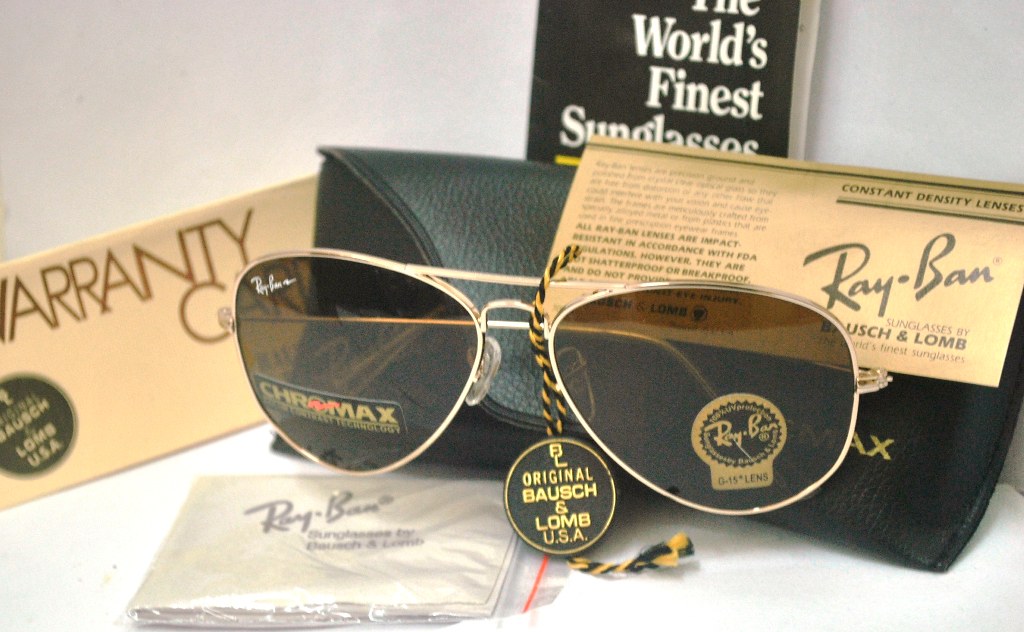This detailed image showcases a meticulously arranged display of Ray-Ban sunglasses and their accompanying items. At the center, a pair of gold-rimmed Ray-Ban glasses prominently feature a circular black tag with gold text labeling them as "Original Bausch & Lomb, USA." The glasses rest partly on a small Ziploc bag containing paper inscribed with "Ray-Ban" in gray, and they lean against a black glasses case.

In the upper right corner of the glasses, a constant-density lens card describes the superior quality of Ray-Ban sunglasses by Bausch & Lomb. To the left of the sunglasses and case, there is a distinctive yellow card with black text indicating it is a Warranty Card. Behind the glasses, a black pamphlet with the white text "The World's Finest Sunglasses" adds a touch of elegance to the display.

Additionally, the lenses have various stickers, including "Ray-Ban" and "Chromex," further highlighting their authenticity and features. A little pendant attached with a black-and-white thread to the center of the glasses reiterates "Original Bausch & Lomb, USA." Overall, the image captures a comprehensive and well-organized presentation of the Ray-Ban sunglasses, their case, and all associated documentation, emphasizing both the product's heritage and high quality.